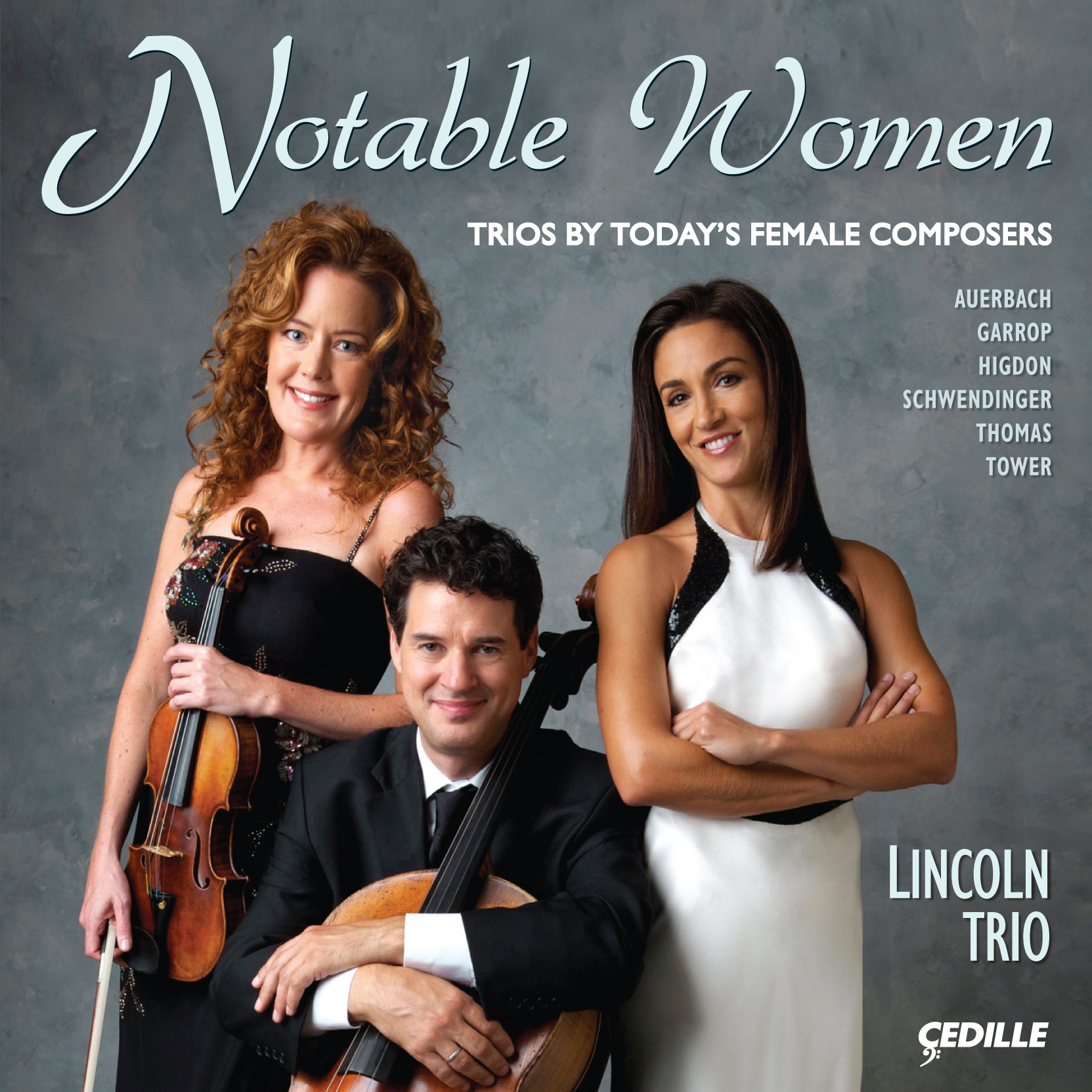This image appears to be the cover of a CD or album titled "Notable Women: Trios by Today's Female Composers." The background is a portrait-style gray, setting a formal and elegant tone. At the top of the cover, the title "Notable Women" is displayed in light blue font, followed by the subtitle "Trios by Today's Female Composers." Along the right side, the names of the composers—Auerbach, Garopp, Higdon, Schwendinger, Thomas, and Tower—are listed.

Prominently featured on the cover are three musicians. On the left stands a white woman with striking red hair, wearing a long black dress with spaghetti straps. She holds a violin and bow, indicating her role as the violinist. On the right, a woman with dark skin and shoulder-length straight brown hair is dressed in a long white gown with black trim. She stands with her hands folded in front, suggesting she might be the pianist or another non-instrumental role within the trio. Seated between them is a white man with black hair, dressed in a suit. He cradles a cello in his arms, reaffirming his position as the cellist.

Toward the bottom right corner of the cover, the ensemble name "Lincoln Trio" is noted, along with the logo and name "Cedille," the record label. The overall composition presents a polished and professional image of the trio, highlighting their collaboration and the notable works of contemporary female composers.